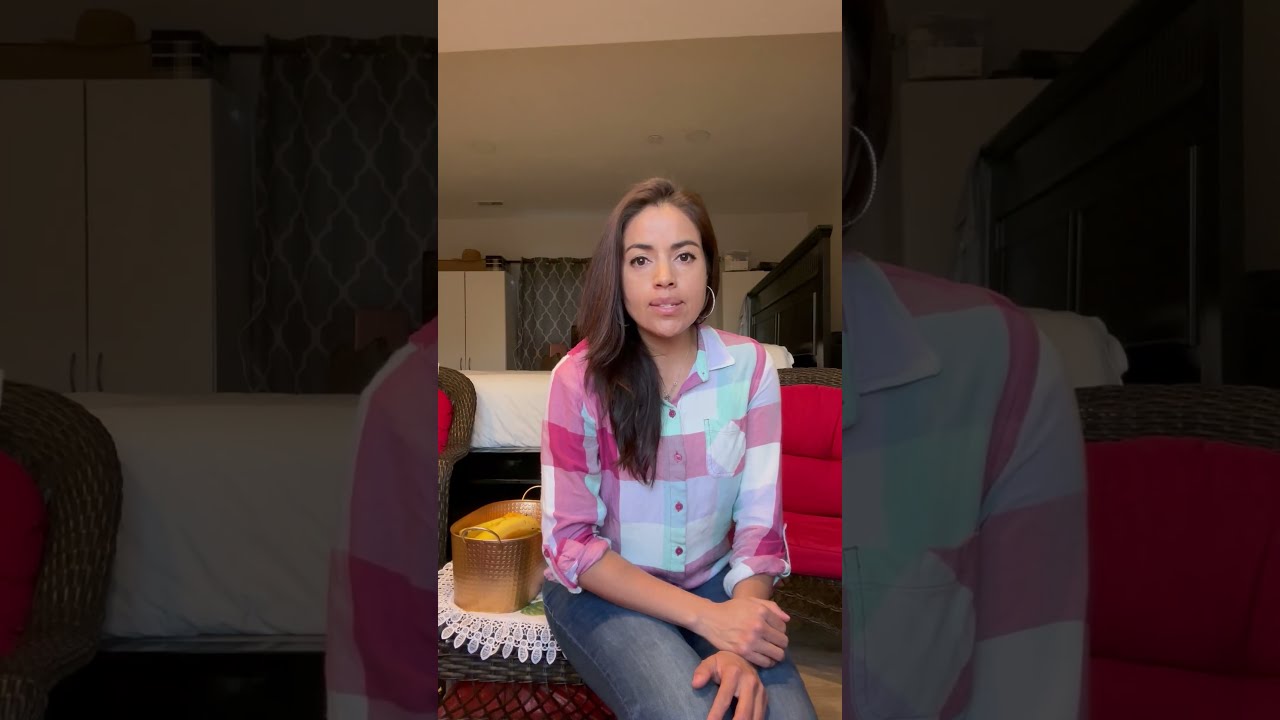In this detailed color photograph, the focus is on a young woman, likely a teenager, seated in an indoor living room. The image is presented in portrait orientation and is centered within an enlarged, darkened landscape orientation frame of the same photo for dramatic effect. The subject has long, dark brown hair draped over one shoulder and is adorned with silver hoop earrings. She is attired in a collared, button-up plaid shirt with a mix of light green, light pink, red, blue, and white squares, the sleeves casually rolled up past her elbows, paired with blue jeans. The woman appears to be grasping her hands in front of her lap and gazing up at the camera, potentially mid-speech, suggesting she may be engaged in a video presentation.

To her left, a gold or bronze-colored basket sits atop a table that she is partially seated on. Behind her, a red upholstered chair and some cabinets are visible, enhancing the cozy living room setting. The background further features a table with a white round tablecloth, more prominently framing the subject with decorative elements such as draperies with a diamond pattern. This composition exudes a sense of photographic realism, capturing the intimate, homely atmosphere of the scene.